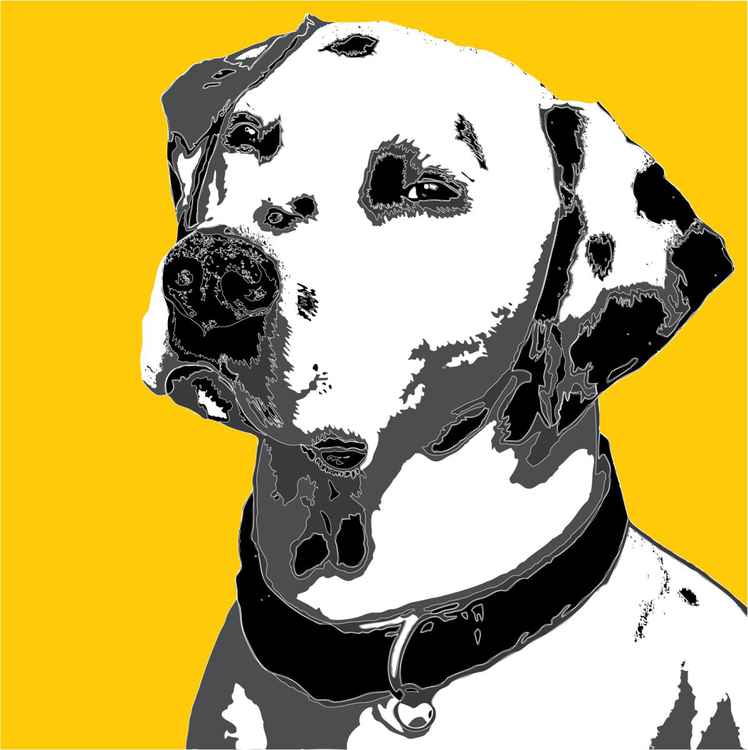In this detailed drawing, a dog—resembling a Dalmatian—sits against a rich, deep yellow background. The illustration showcases the dog from just below the shoulders upward, focusing primarily on its face and neck. The dog's head is slightly tilted, giving it an inquisitive look, with closed mouth and expressive, squinting eyes. The dog’s fur is predominantly white, accented by black spots, particularly noticeable on its ears, under its chin, and around its eyes. Its nose is black, complementing the black collar it wears, which features a typical buckle and something hanging from the front. The dog gazes directly at the viewer, capturing their attention with its direct, engaging expression.